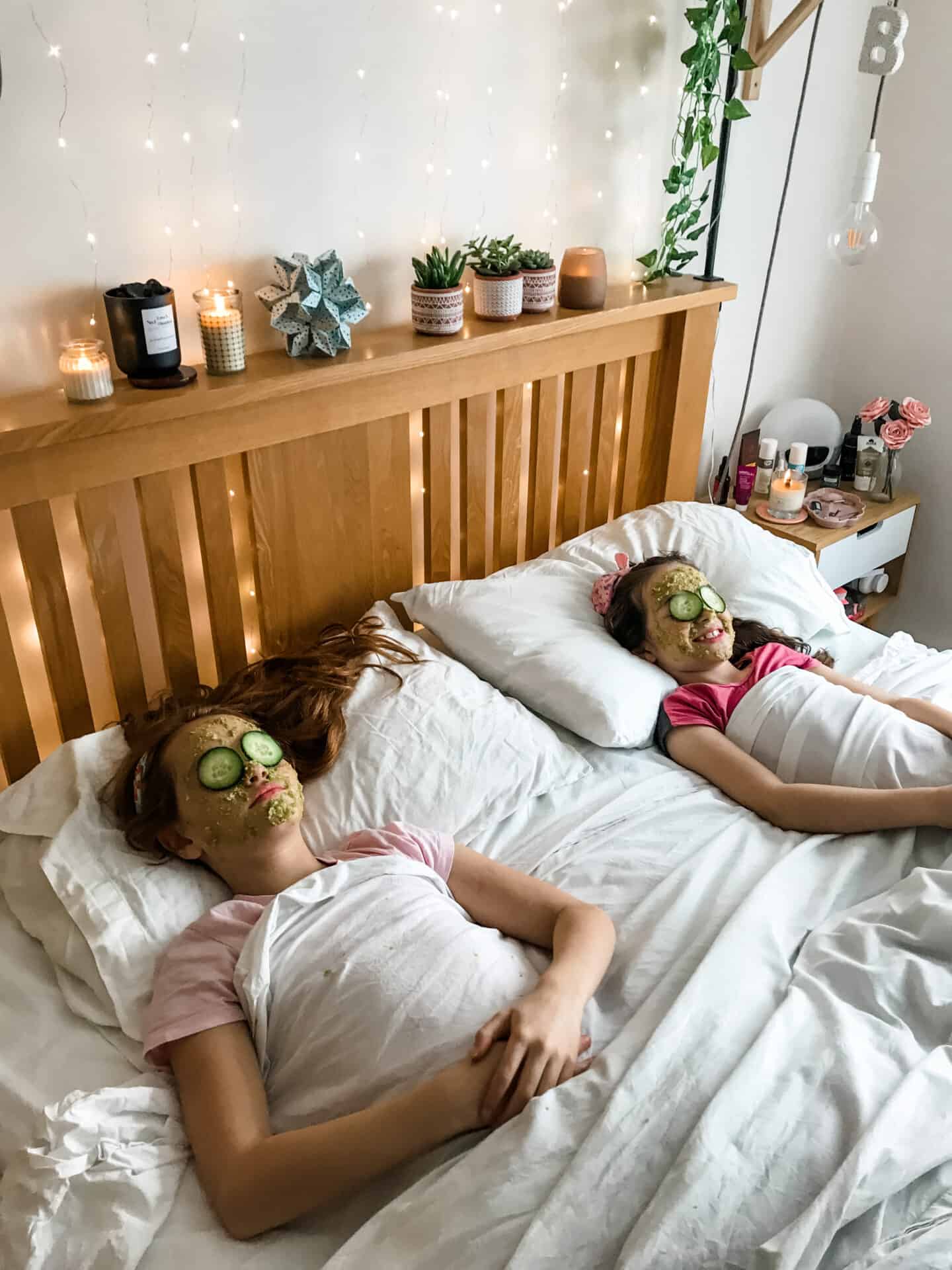The photograph depicts a cozy bedroom scene, showcasing two Caucasian girls, approximately 10 years old, lying side by side in a shared queen-sized bed adorned with crisp white sheets and pillows. The bed, featuring a brown wooden headboard with vertical slats, adds a rustic charm to the room. Above the headboard, several jar candles are lit, infusing the air with their likely soothing scents, alongside various potted succulents and a vine plant that trails down the white wall in the top right corner. 

The girls, seemingly enjoying a spa day, are both wearing pink short-sleeve shirts and green face masks, complete with cucumber slices over their eyes. The girl on the left appears to be in a deeper state of relaxation, while the girl on the right, with a smile, engages with the camera. Their arms rest gently atop the sheets that cover them up to their chests. 

Beside the bed stands a small side table featuring a light-colored wooden top and sides with a white drawer. The table is adorned with a vase of three roses, numerous bottles, and another lit scented candle, creating a serene and inviting atmosphere. The overall image exudes a peaceful, intimate moment, capturing a blend of youthful fun and relaxation in a homely setting.